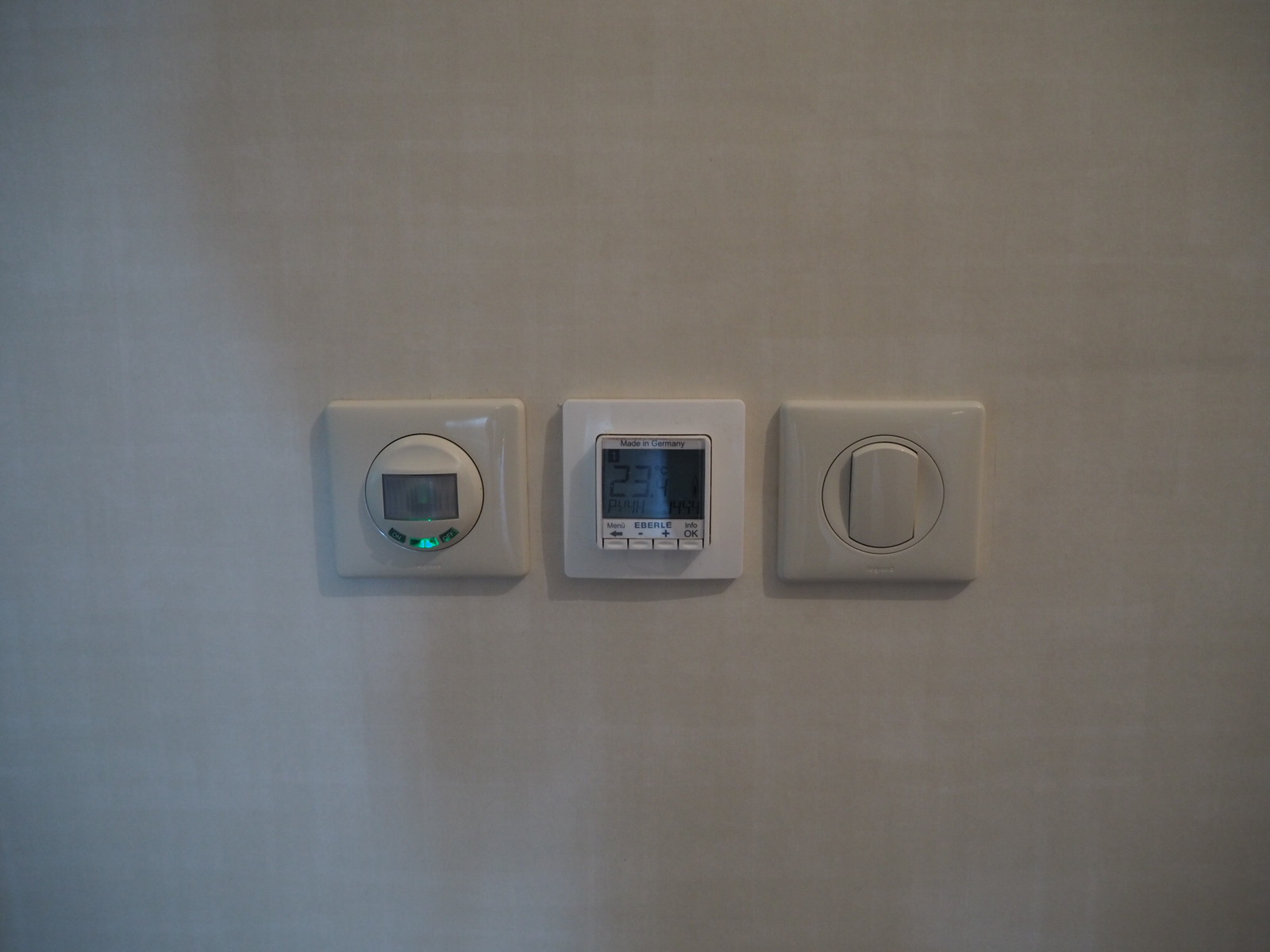This detailed caption describes a photograph of a section of a beige wall featuring home control devices. Three square fixtures are arranged horizontally. The fixtures on the left and right are made of tan-colored plastic, while the one in the center is white.

The left fixture contains a circular display with a clear window, likely for reading measurements. Inside this circular display are indicator lights, with one light illuminated in a light blue hue.

The central fixture is white and measures approximately four to five inches in height and width. It houses a small screen displaying digital numbers, situated at the top half of the square. Below the screen are several control buttons.

The right fixture is similar to the left, made of tan-colored plastic, featuring a circular component within it. Within this circle is an almost-rectangular, vertical beige knob.

The arrangement and details suggest that these are home control devices, possibly for lighting, temperature, or other residential systems.